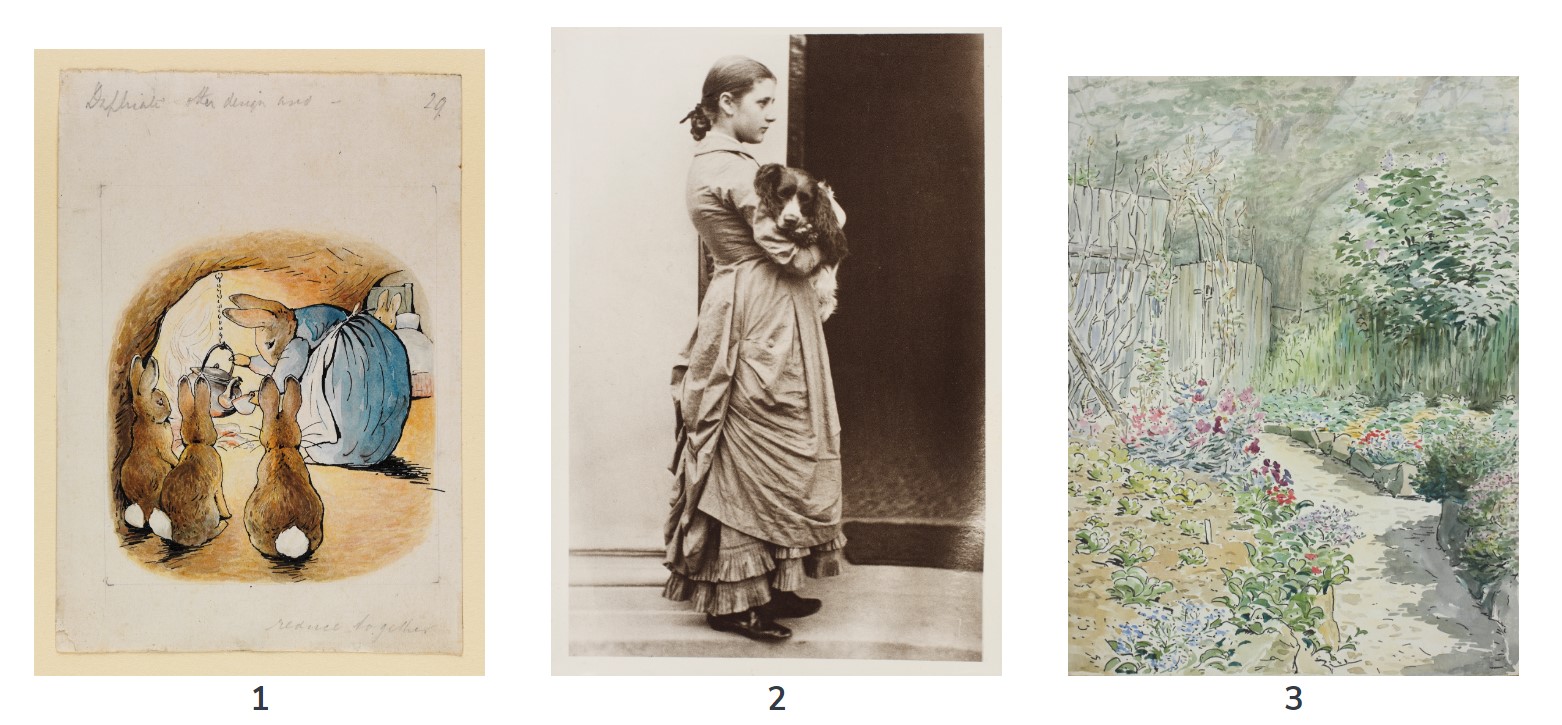This image features three distinct sections, each showcasing a different scene, labeled with numbers. On the far left (labeled number one) is an illustration of a mother rabbit in a blue, 19th-century style dress, pouring tea from a kettle. She is observed by three younger brown rabbits with white tails. The scene has a yellow border and a brown background, with additional rabbits faintly visible in the distance.

The middle section (labeled number two) displays an old sepia-toned photograph of a young woman in a long dress, holding a cocker spaniel. She has short, brown hair and black shoes, and the setting appears to be indoors.

On the far right (labeled number three) is a watercolor painting of an outdoor scene featuring a concrete or cobblestone walking path that leads up to a gated area, possibly the entrance to a backyard. Surrounding the path are green plants, various colorful flowers, and trees, with a noticeable tree in the far distance.